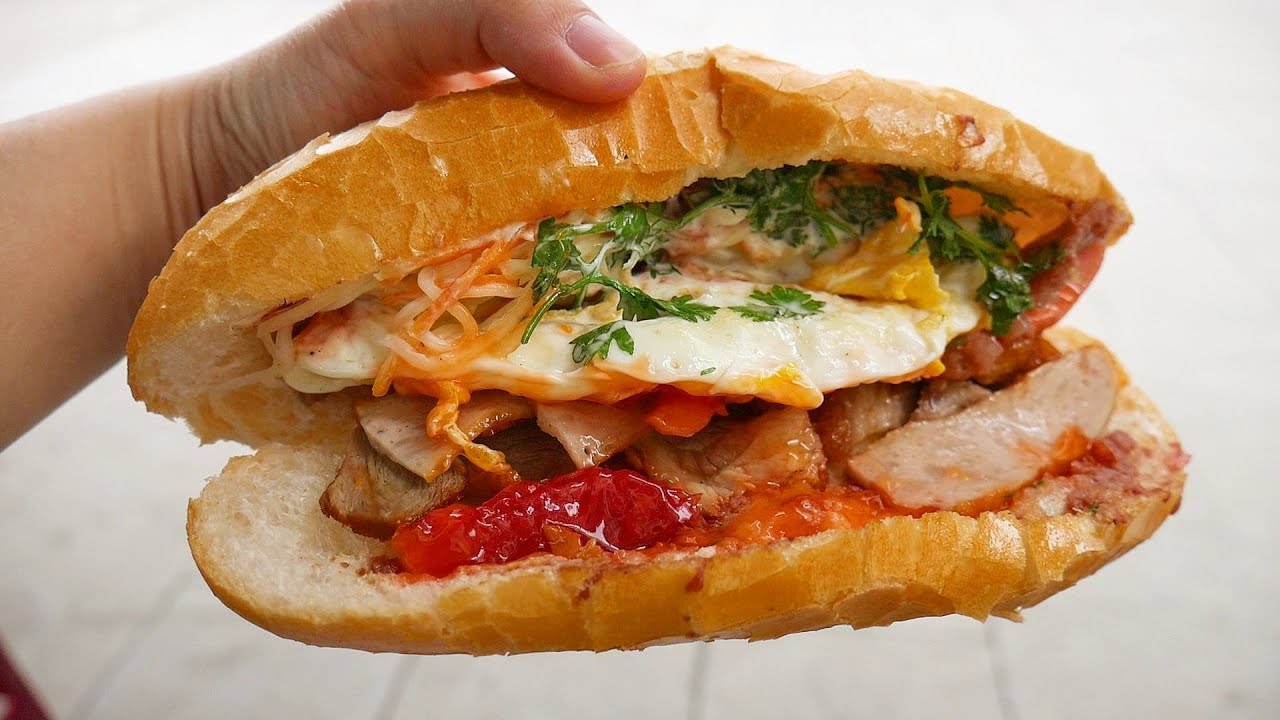In this detailed image, we observe a Caucasian hand, likely belonging to a young man, gripping an open, decently long baguette sandwich from the left side, allowing us to view its contents clearly. The background, a white tile floor, features faint lines adding minimal texture. The sandwich displays a colorful and generously stuffed interior, with ingredients from top to bottom: starting with a layer of brownish string-like noodles or grated cheese, followed by fresh green cilantro, and what appears to be slices of mozzarella cheese. There’s a noticeable section of yellow mustard, giving a hint of tanginess. Beneath the cheese, there are pieces of brownish-colored chicken and what looks like slices of turkey or possibly ham, interspersed with vibrant red pepper or red sauce. The lower part of the sandwich contains more brownish meat, potentially meatballs, firmly embedded in the white bread, which looks slightly soggy. The sandwich is packed to the brim, with ingredients nearly spilling out, especially from the edges, where noodles and cilantro are precariously close to falling.